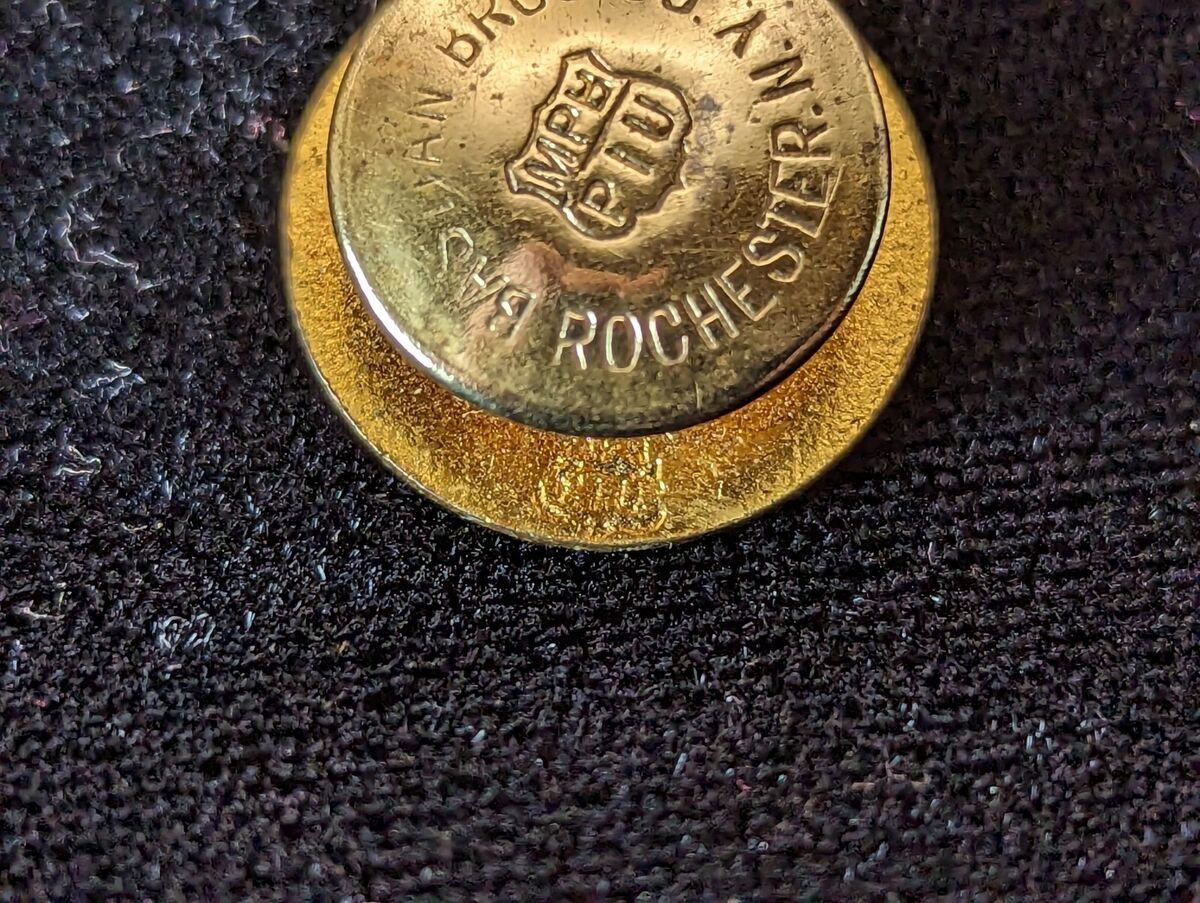This close-up macro photograph showcases a weathered, metallic button or pin with a vintage appearance, resting on a piece of black fabric. The shiny gold or brass object features a detailed emblem in the center that reads "MPH" at the top and "PIU" at the bottom, resembling a police badge or official insignia. Surrounding the emblem, partially rubbed-out text is inscribed, with "Rochester NY" clearly visible along the bottom edge, suggesting a connection to Rochester, New York. The button, which has seen significant wear with numerous scuff marks, is placed on a tightly woven, soft-textured black material, possibly tweed, with strands of dust or hair visible on its surface.